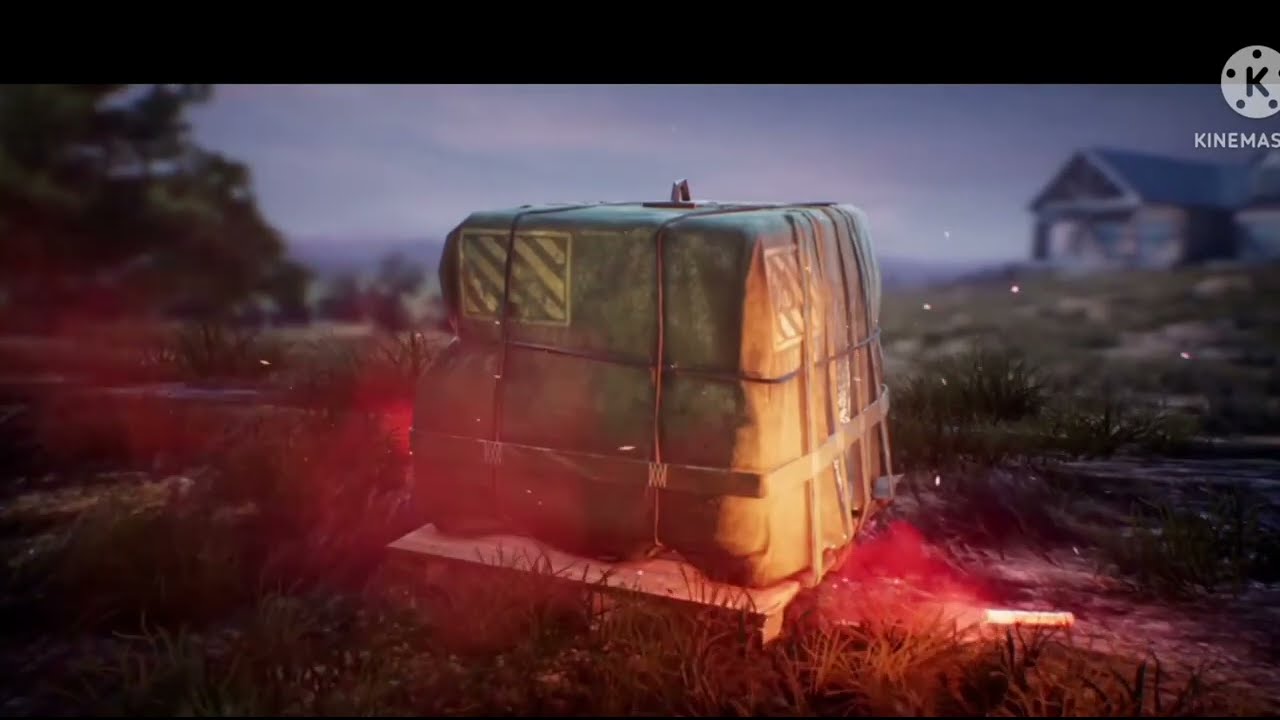The image is a horizontal rectangular screenshot taken from a video game, likely PUBG. In the foreground, there is a central focal point: a large rectangular drop package covered with a green cloth and secured with brown straps, which appear meticulously tied down. The drop sits atop a short wooden platform, and it features alternating black and yellow diagonal lines on its sides, suggesting military or cautionary tagging.

Surrounding the drop is a striking red smoke effect, indicating recent deployment or impact. The ground is grassy and green, extending to the background, which gradually blurs. To the right in the blurred background, a wooden house with a hipped roof is visible, while the left side of the image features large tree branches with green leaves. The sky overhead is a bluish-gray, resembling an early evening setting.

At the top right corner of the image is a slightly cut-off watermark featuring the capital letter "K" inside a white circle, accompanied by the text "KINDMASTER" in white capital letters. A thick horizontal black strip runs across the top of the image, adding a distinct border.

Overall, the detailed elements suggest a dynamic and immersive scene from the video game, capturing the moment of a fresh supply drop in a lush, slightly hazy environment.